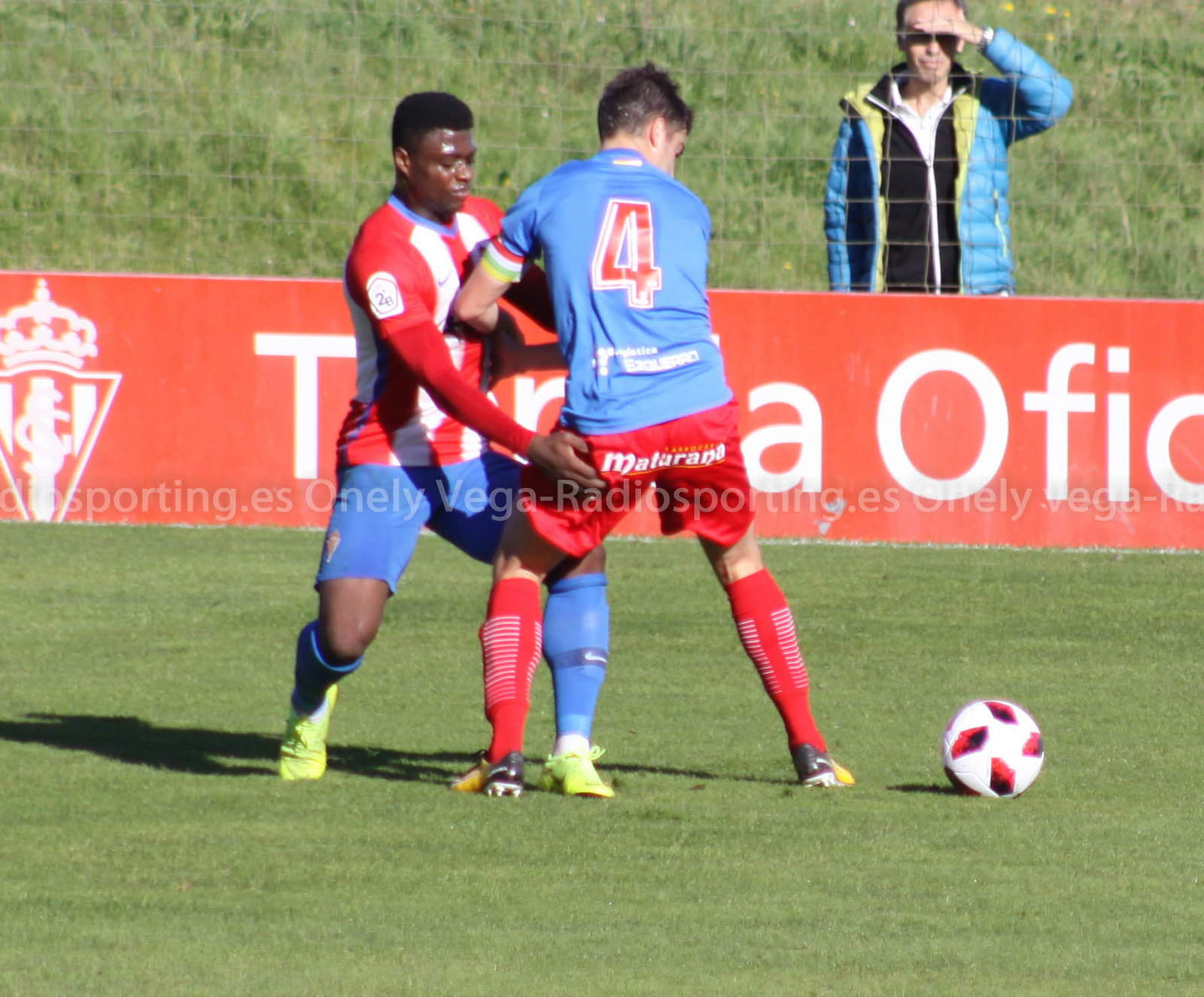In the dynamic scene depicted, two soccer players are intensely vying for control of a soccer ball positioned to the right of them. The player on the left is an African man dressed in a striking red jersey with white stripes running down the chest, blue shorts, and greenish shoes. His dark hair is thick and voluminous. He reaches towards the other player, emphasizing physical engagement and competition. The player on the right is a white man with short black hair. He is clad in a blue jersey featuring the number 4 on the back, complemented by red shorts and red shin guards.

The background sets a vivid stage with a red banner stretching horizontally from left to right. A notable tower-like structure anchors the left end of the banner, with the partially obscured text revealing a visible 'T' at the start and an 'A' at the end, suggesting part of a larger word. Adjacent to this, another word begins with letters that could be "O-F-I-C" or something similar, partially concealed. Above this scene, a thin metal fence separates the field from the spectators, where a person, possibly a coach, is seen shading their eyes with their right arm. This individual, wearing sunglasses, is distinguishable by their layered attire: a blue outer jacket, a black inner jacket, and a white collared shirt underneath.

Adding a further touch of realism, a watermark reading "theradiosporting.es" is subtly imprinted on the image, marking its source. This detailed and vibrant scene captures the intense focus and physicality of the sport, set against a lively backdrop that underscores the event's atmosphere.